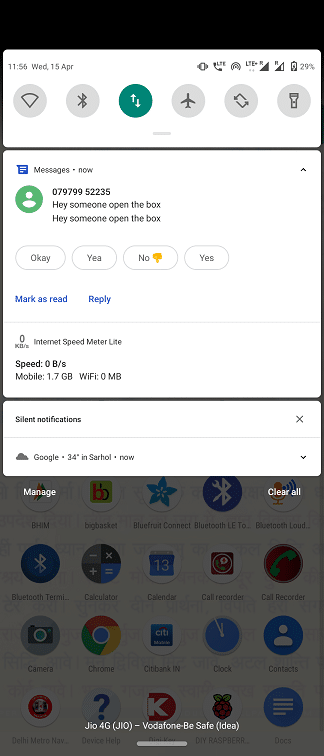This image is a screenshot of a smartphone display, showcasing a predominantly white background with a standard array of interface elements. At the top of the screen, various icons are present, including the LTE connectivity indicator and additional small icons reflecting network status. A battery icon positioned at the top-right corner displays 29% battery life remaining. 

Beneath this top section, a horizontal row features six selectable buttons, with one button highlighted in green to denote its active status. Following this, a section dedicated to messages appears, capturing an ongoing text conversation. Further down, there's a compact segment labelled "Internet Speed Meter Lite," presenting current speed metrics along with mobile and Wi-Fi information.

An additional field is discernible below this, labeled as a "Silent Notifications" option, though it is currently not selected. A comment regarding Google information is noted beneath, leading further down to an apps page. This page exhibits a colorful array of various application icons, each clearly labeled with the app’s name and function. 

At the very bottom of the screen, the text reads: "Geo4G, GIO, Vodafone, Be Safe."